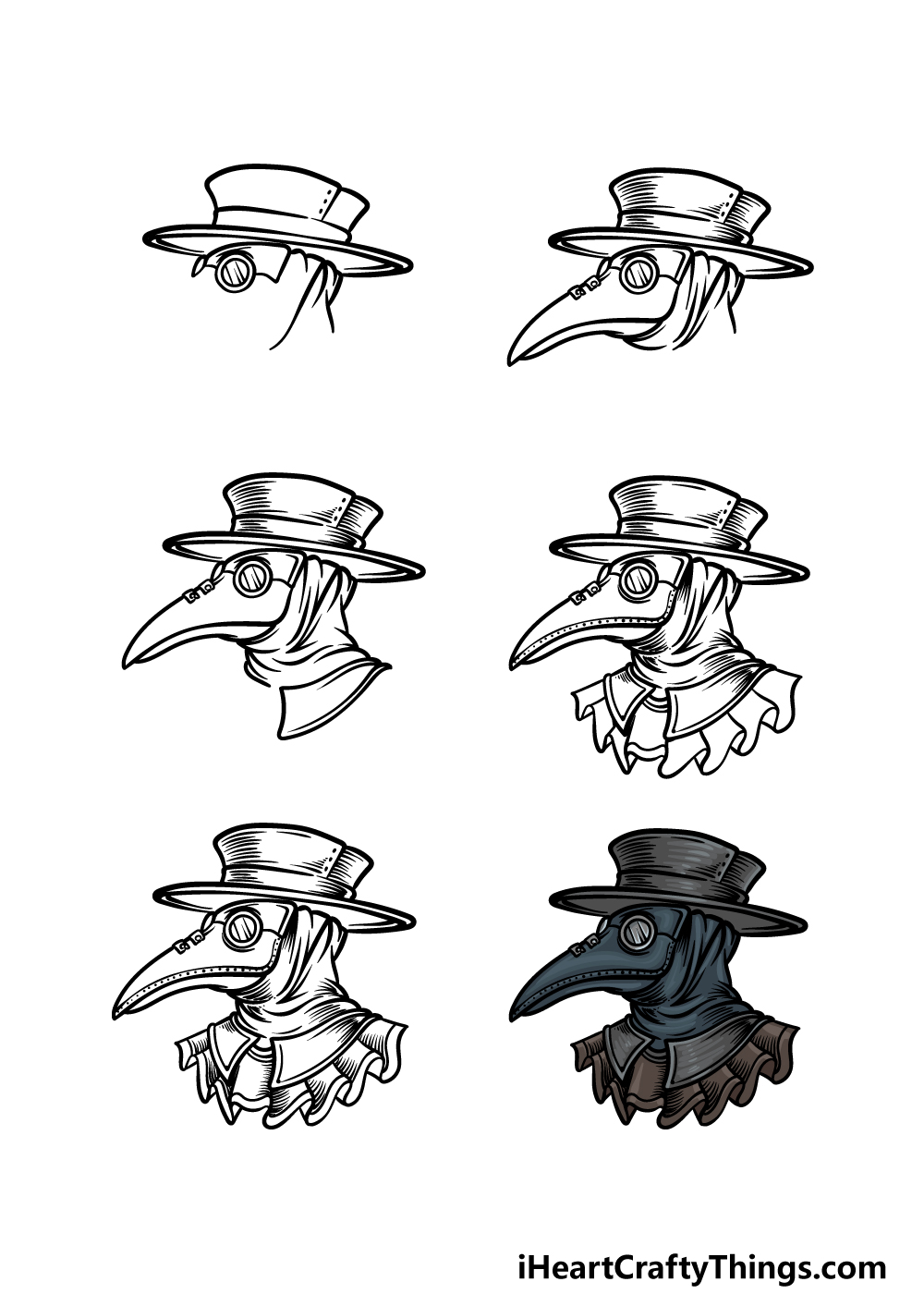The image consists of a series of six illustrations arranged in a 2x3 grid, depicting the progressive stages of creating an elaborate raven mask, reminiscent of those used during the Plague years. Starting from the upper left, the initial sketch shows the faint beginnings of a black pencil drawing on a white background, highlighting a partial face and a hat that resembles a beak-like mask. The upper right advances the sketch to almost a complete line drawing, now featuring more facial details including an eye and a chin strap. 

In the middle left, the drawing begins to include the collar, which is frilled and in shades of brown and gray. The middle right further refines the illustration, nearly completing the line art with additional intricate details. By the lower left, the line drawing is fully detailed, ready for coloring. The final image in the lower right presents the fully colored mask, portraying a dark blue headpiece, a gray to almost black hat, and shaded facial features giving the mask a bird-like appearance. The collar's delicate frills remain brown and gray, completing the eerie yet fascinating raven mask illustration. At the bottom of the image, the website "iheartcraftythings.com" is displayed, suggesting the source of this artistic guide.